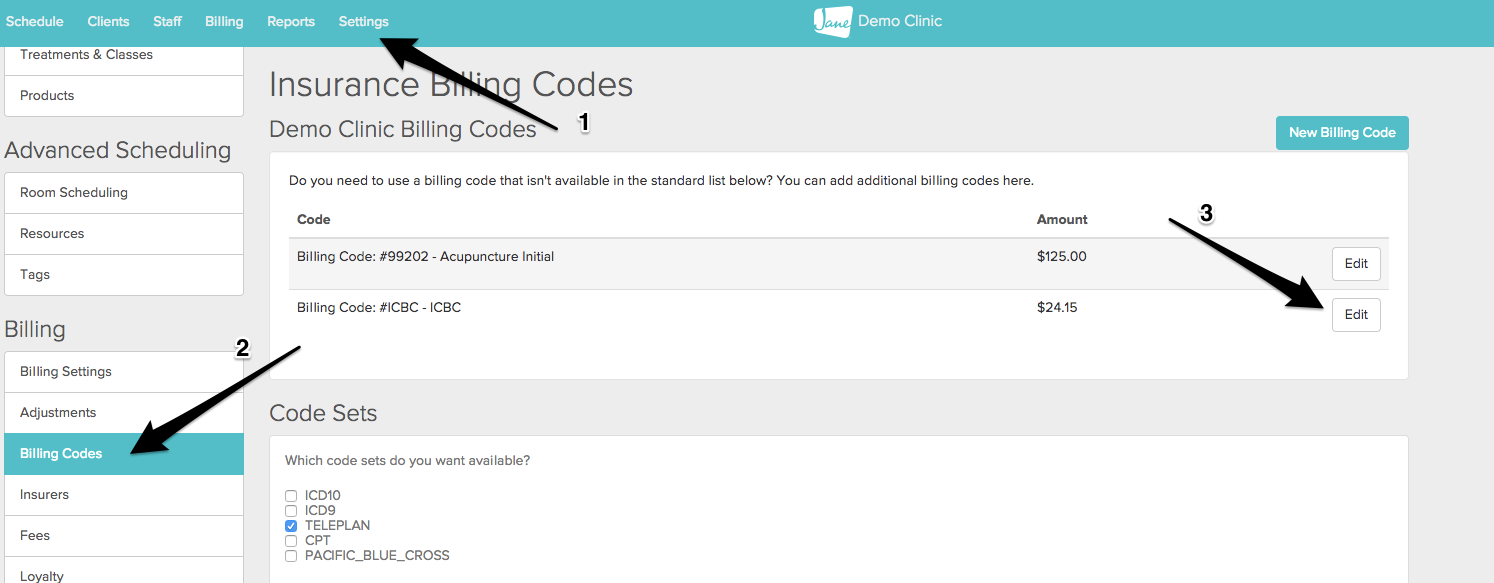Here's a cleaned-up and detailed caption for the described image:

"This image depicts a web page titled 'June Demo Clinic' with a main header that reads 'Insurance Billing Codes, Demo Clinic Billing Codes.' On the left side of the page, there is a vertical list of headings which includes: Room Scheduling, Resources, Tags, Billing, Billing Settings, Adjustment, Billing Codes, Insurers, Fees, and Loyalty. To the right of this list, there are several checkboxes corresponding to various code sets. The options available are ICD-10, ICD-9, Teleplan (which is checked and marked with a blue tick), CPT, and Pacific Blue Cross. Additionally, the page displays example prices and amounts alongside their respective billing codes, suggesting that it serves as a tutorial for understanding and navigating insurance billing codes."